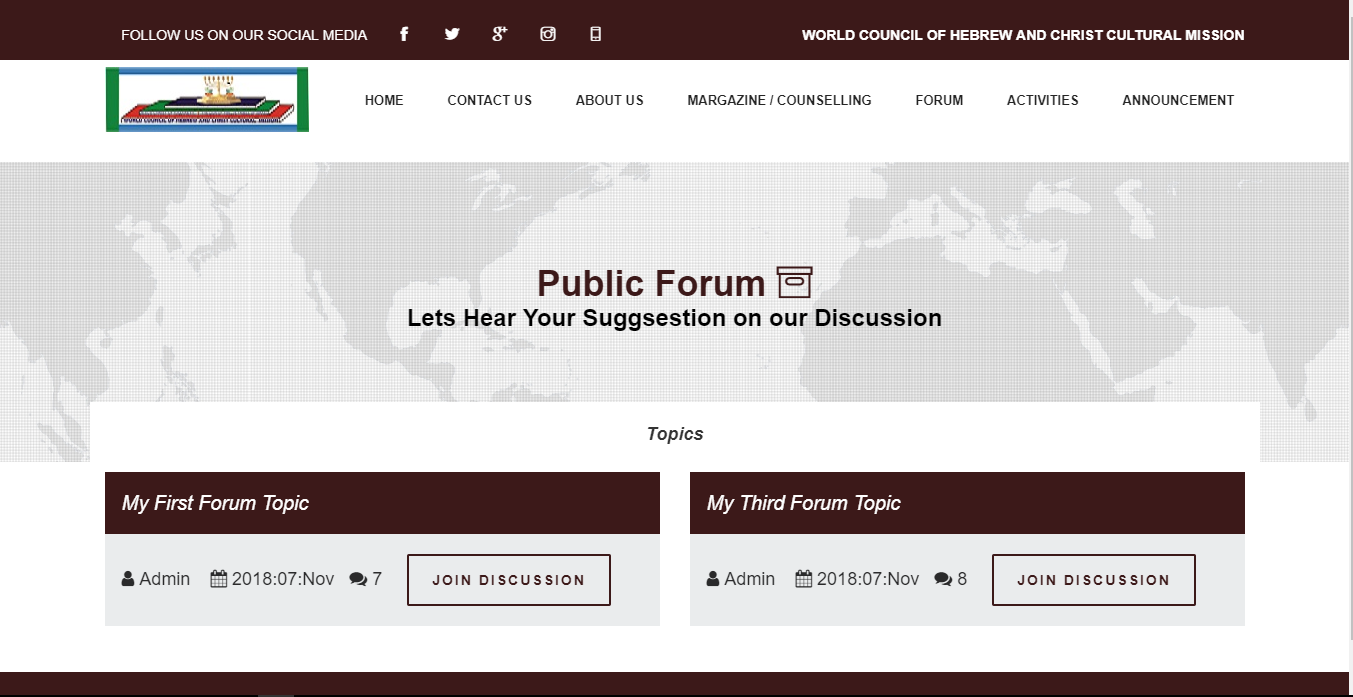A screen capture of a webpage features a detailed layout and various design elements. At the very top, there is a navigation ribbon with options such as Home, Contact Us, About Us, Magazine, Counseling, Forum, Activities, and Announcements. Below this, another horizontal ribbon starts at the upper left corner, displaying the message "Follow us on social media" with icons for Facebook, Twitter, Google Plus, and Instagram.

In the left part of this second ribbon, there is a colorful menorah icon, adding a splash of color to the predominantly gray and white page. To the right of the menorah icon, the header reads: "World Council of Hebrew and Christ Cultural Mission."

Below these ribbons, a light gray patterned background depicts the seven continents. Superimposed on this background is the bold title "Public Forum" accompanied by a subtitle that reads "Let's hear your suggestions on our discussion."

Further down, there is a rectangular white section labeled "Topics." On the left side of this section, one topic is titled "My First Forum Topic," moderated by "admin" with a date of "2018, 07 November" and marked with seven comments. On the right, another topic reads "My Third Forum Topic," also moderated by "admin" with the same date but showing eight comments.